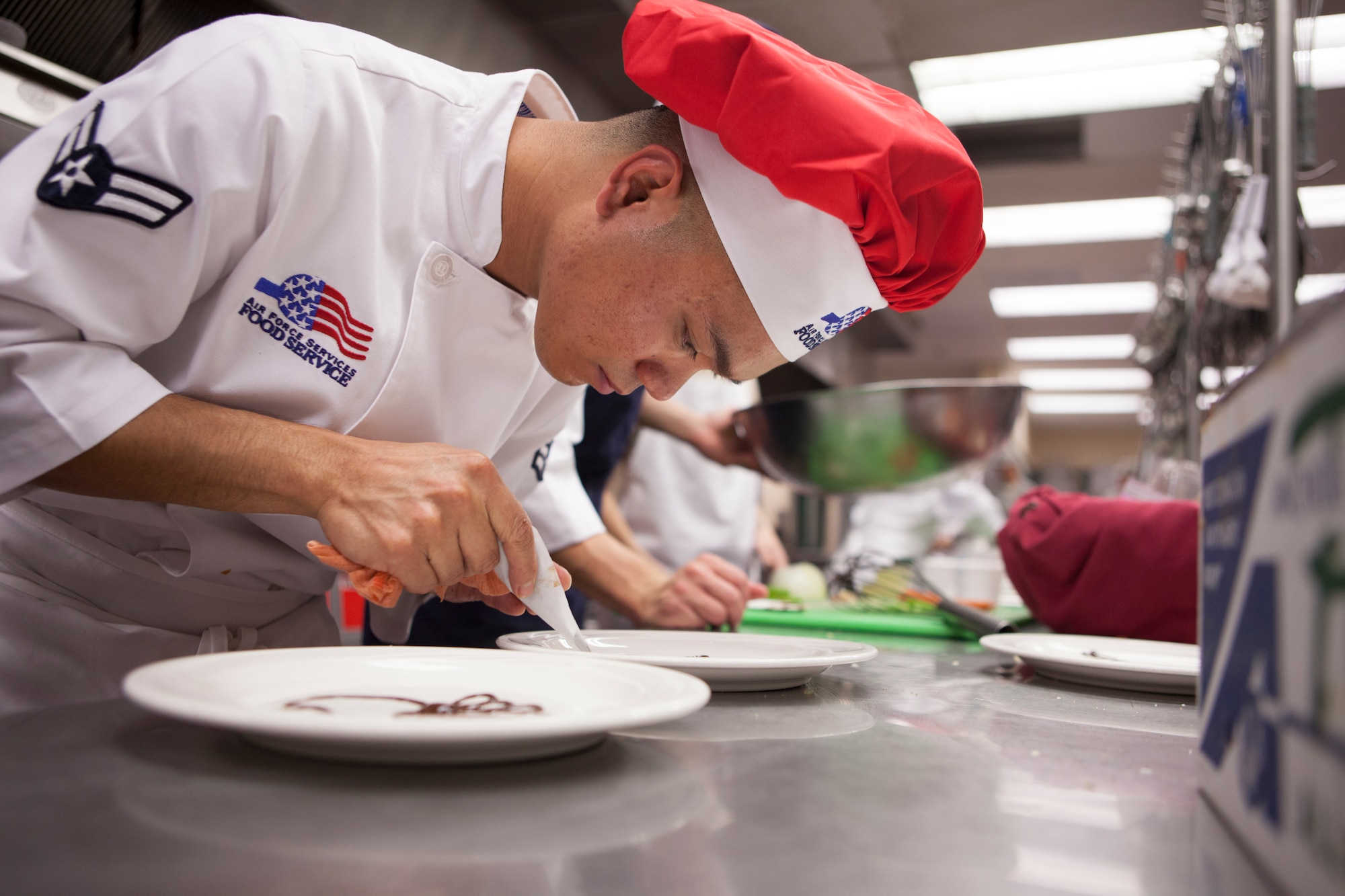In this landscape photograph, we see a close-up of an Asian male chef with semi-dark skin, deeply engrossed in preparing a dish. He is wearing a red chef's hat with a white trim, emblazoned with the emblem "Air Force Services Food Service," which matches the emblem on his white coat. His coat also displays an American flag logo and a distinctive star badge on his right upper arm, indicative of his association with the U.S. Air Force Food Service. The chef is hunched over a marble countertop, meticulously using a piping bag to apply sauce or icing onto a plate. Next to him is another plate featuring piped chocolate. The background reveals another chef, holding a large silver bowl, and a cutting board with orange vegetables and a knife, all set within a brightly lit kitchen illuminated by numerous fluorescent lights.